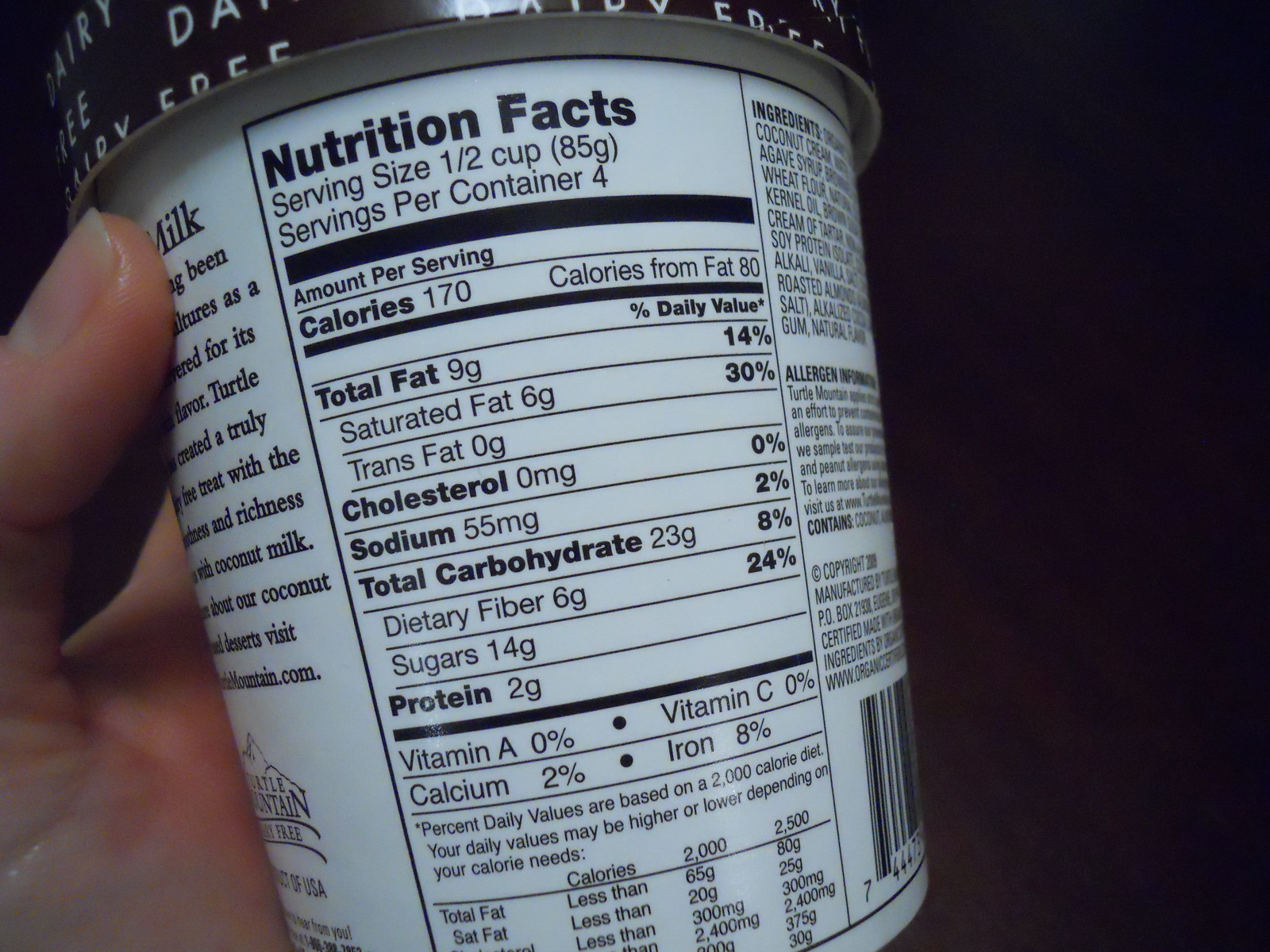This color photograph captures a close-up of a person's left hand holding a pint-sized ice cream carton, with the hand positioned at the bottom left and only the side of the thumb visible. The carton is primarily white with a dark brown rim around the black lid, adorned with partially readable white letters along the edge, including the term "dairy-free." The carton’s front is turned away from the viewer, obscuring the brand name and flavor, but revealing detailed nutritional information on its back.

Prominently displayed in black letters are the words "Nutrition Facts," followed by specific details: Serving size 1/2 cup (85g), servings per container 4. The nutrition breakdown for each serving is as follows: 170 calories, 80 calories from fat, 9 grams of total fat, 6 grams of saturated fat, 0 grams of trans fat, 0 milligrams of cholesterol, 55 milligrams of sodium, 23 grams of total carbohydrates, 6 grams of dietary fiber, 14 grams of sugars, and 2 grams of protein. The vitamins and minerals content is - Vitamin A: 0%, Vitamin C: 0%, Calcium: 2%, Iron: 8%. These percentages are based on a 2,000 calorie daily diet.

Additionally, a part of the UPC code is visible on the right edge, while on the left side, there is a partially visible paragraph providing a description of the product, accompanied by a logo resembling a mountain. The overall setting focuses on the functional elements of the carton, emphasizing its nutritional information and indicating it is a dairy-free product, presumably ice cream, based on context clues and visible ingredients.